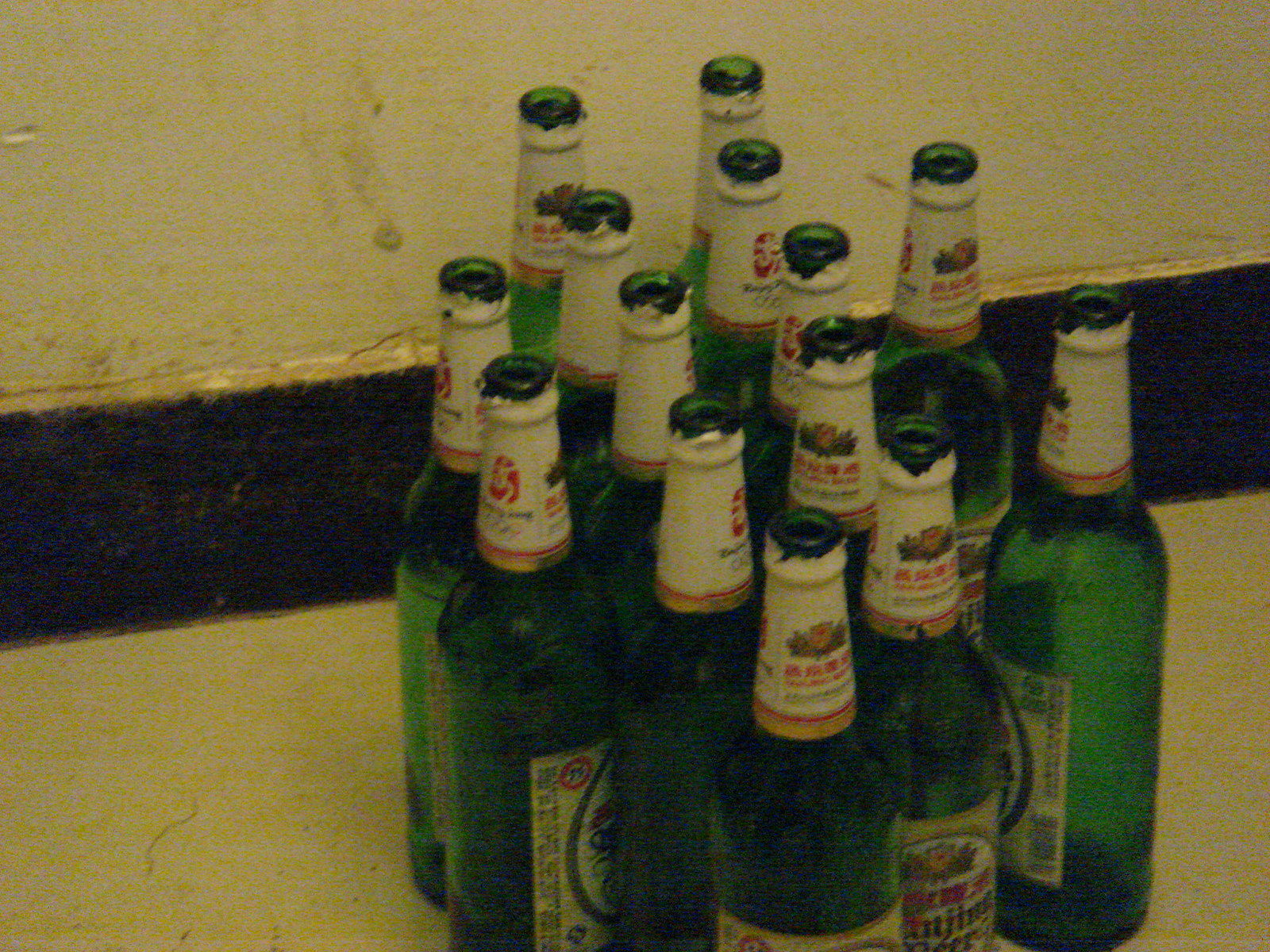In this dim, fuzzy photograph, we observe 14 identical glass beer bottles, all of a green hue and transparent, positioned together in a tattered, raggedy corner. The background features a very dirty, off-white wall with prominent dark and yellow-brown stains, partially obscured by a white surface likely made of concrete, which extends from the floor and includes a black trim. Each bottle, now open and empty, exhibits a white label around its neck adorned with red writing, possibly depicting a lion or a similar symbol, and various forms of ripped paper or aluminum neck coverings. The front label on some bottles is yellow with a white circle, showcasing more red and black text along with a crest-like emblem, potentially surrounded by floral imagery. A barcode is visible on one bottle, and the language on the labels appears to be either Japanese or Chinese. This cluttered assembly of bottles, captured in a low-quality, pixelated image, hints at their abandonment and potential for recycling.